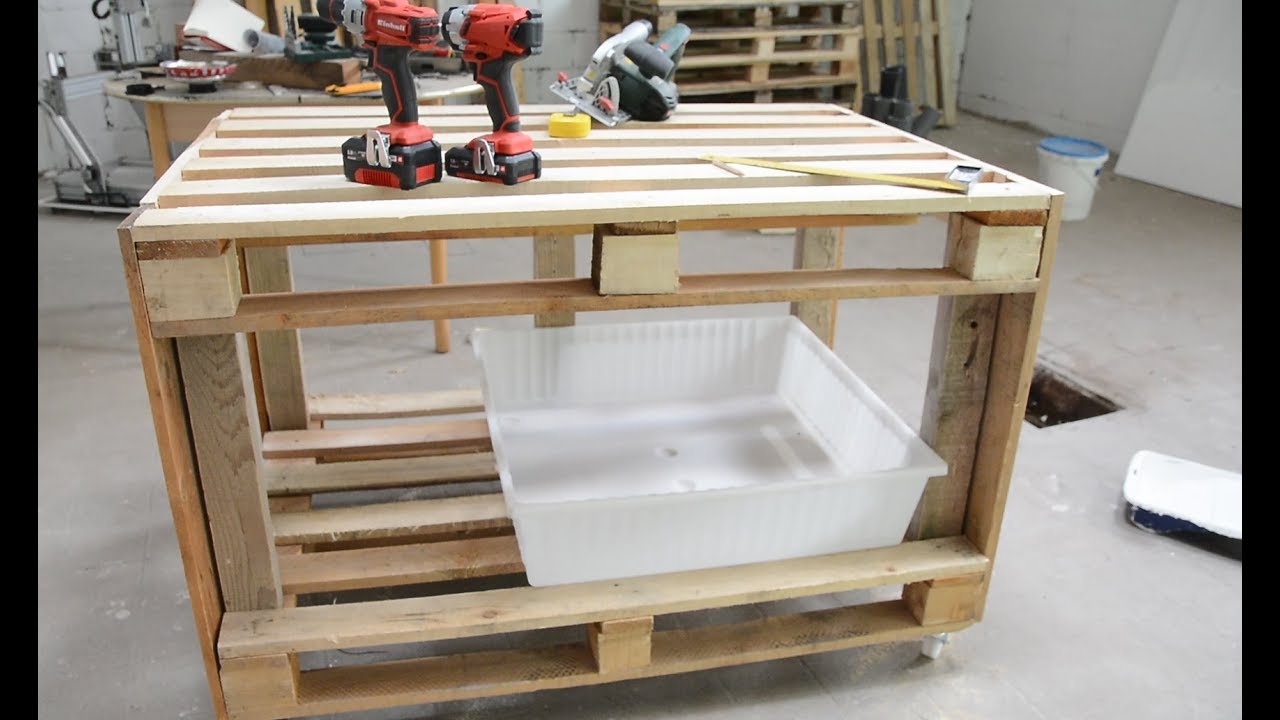The image depicts a woodworking workshop with a concrete floor and unfinished white and gray walls. In the center of the space stands a large handmade workbench, fashioned from recycled wooden pallets, featuring added wooden supports for structural integrity. The table has an additional board on the left side for extra stability. On its top shelf, two red battery-operated handheld drills are positioned upright, accompanied by a handsaw and a yellow measuring tape. Below, a translucent frosted plastic bin is visible on the lower shelf. The background reveals several stacked pallets leaning against the wall and another cluttered table filled with various tools and equipment, including what appears to be a jack. The workbench, possibly part of an ongoing project that could serve as the base for cabinets or a mobile kitchen island, showcases the workshop's industrious atmosphere.